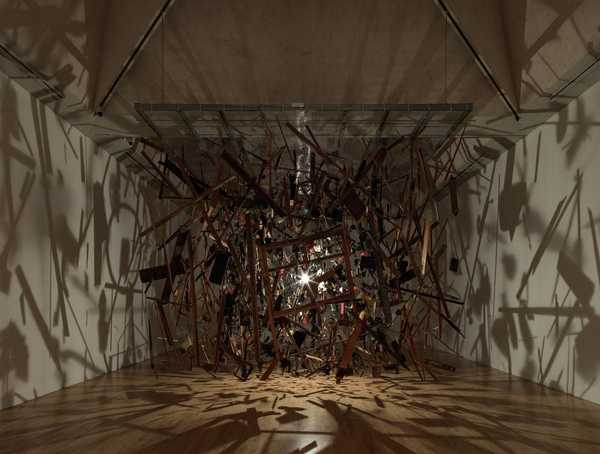The image captures an art installation centered in a long room with light gray walls and brown hardwood floors. The centerpiece of the installation appears as a chaotic yet artistic explosion made up of numerous twisted and linear metal bits in black, bronze, and brass colors. A prominent light source located in the center casts dynamic shadows on all surrounding surfaces, including the floors and walls, creating an intricate interplay of light and shadow. Overhead, some cables contribute to the complex visual scene. The overall effect is an illusion of movement and depth, where the light filters through the metal elements, casting elongated and fragmented shapes across the room.